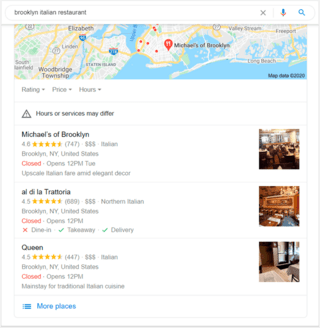The image depicts a search for "Brooklyn Italian restaurant," as seen in the text within the search bar. Positioned to the right of the search bar are an 'X' to delete the text, a microphone icon for voice input, and a blue magnifying glass icon indicating the search function.

Central to the image is a map highlighting various locations, with a prominent orange pin marked with a fork and spoon icon denoting 'Michaels of Brooklyn.' Surrounding this primary pin are numerous smaller pins or dots indicating other restaurants or points of interest in the area. The map includes regions like Woodbridge Township, Elizabeth, New Jersey, and Staten Island. 

Below the map, there are dropdown menus for filter options such as rating, price, and hours. An exclamation mark within a triangle warns that hours or services may differ.

The first search result is 'Michaels of Brooklyn,' boasting a rating of 4.6 out of 5 stars from 747 reviews. It features three dollar signs ($$$), suggesting it is somewhat pricey. The restaurant is described as an upscale Italian establishment with elegant decor. At the time of the search, it was closed and scheduled to open at 12 p.m. on Tuesday. A photo on the right side shows a bright and airy dining area with numerous tables.

The second result is 'Al Di La Trattoria,' rated at 4.5 out of 5 stars with 689 reviews. It also carries three dollar signs ($$$) and specializes in Northern Italian cuisine. Located in Brooklyn, this restaurant was also closed at the time of the search and was set to open at 12 p.m. Unlike the other options, it offers only takeaway and delivery services, with a corresponding restaurant image on the right.

Lastly, the third result is 'Queen,' with a rating of 4.5 out of 5 stars from 447 reviews, also denoted by three dollar signs ($$$). It is a staple for traditional Italian cuisine in Brooklyn. Like the others, it was closed during the search and due to open at 12 p.m. The accompanying image captures the entranceway of the restaurant.

At the bottom of the search results, an icon with three dots and three lines suggests there are more places to explore.